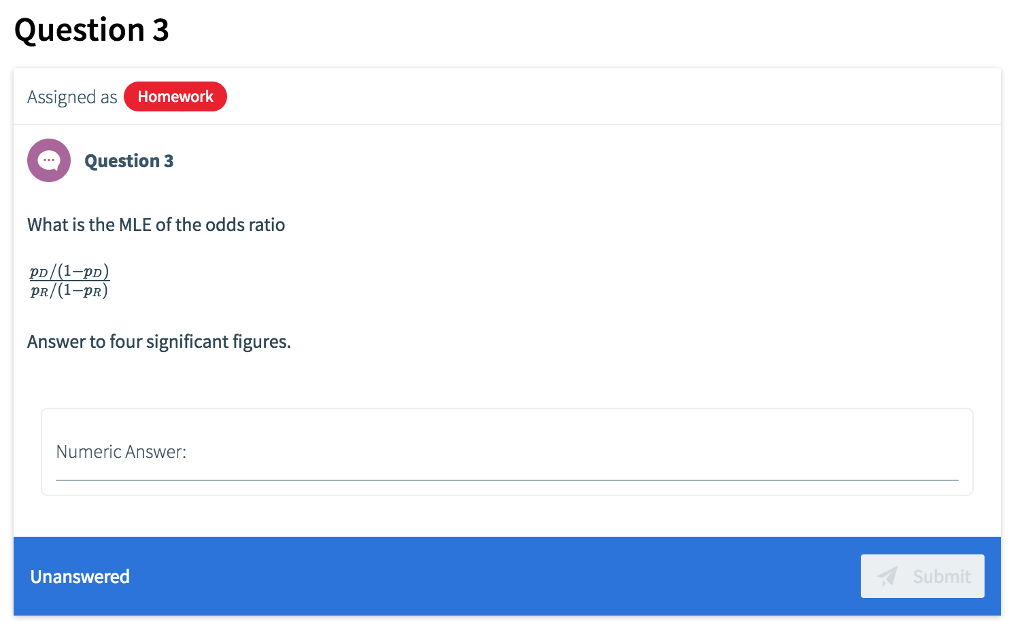At first glance, the image appears to be a web page displaying a homework assignment. At the very top, in bold, black lettering, it reads "Question 3," with a capital Q and the rest of the word in lowercase. Below this heading, there is a rectangular box. At the top of the box, "Assigned As" is written in blue text, followed by a red tab labeled "Homework" in white letters.

A horizontal line divides this section from the content below. On the left-hand side, just below the dividing line, there is a purple circle containing another smaller circle with three dots inside. Adjacent to this icon, it states "Question 3" again. 

The question itself is written in blue text below this section, asking, "What is the MLE of the odds ratio?" Following the question, there is an arithmetic formula presented. It reads, in capital letters, "PD / (1-PD)," and below a separating line, it continues with "PR / (1-PR)." This formula appears to be the mathematical expression required to solve the problem.